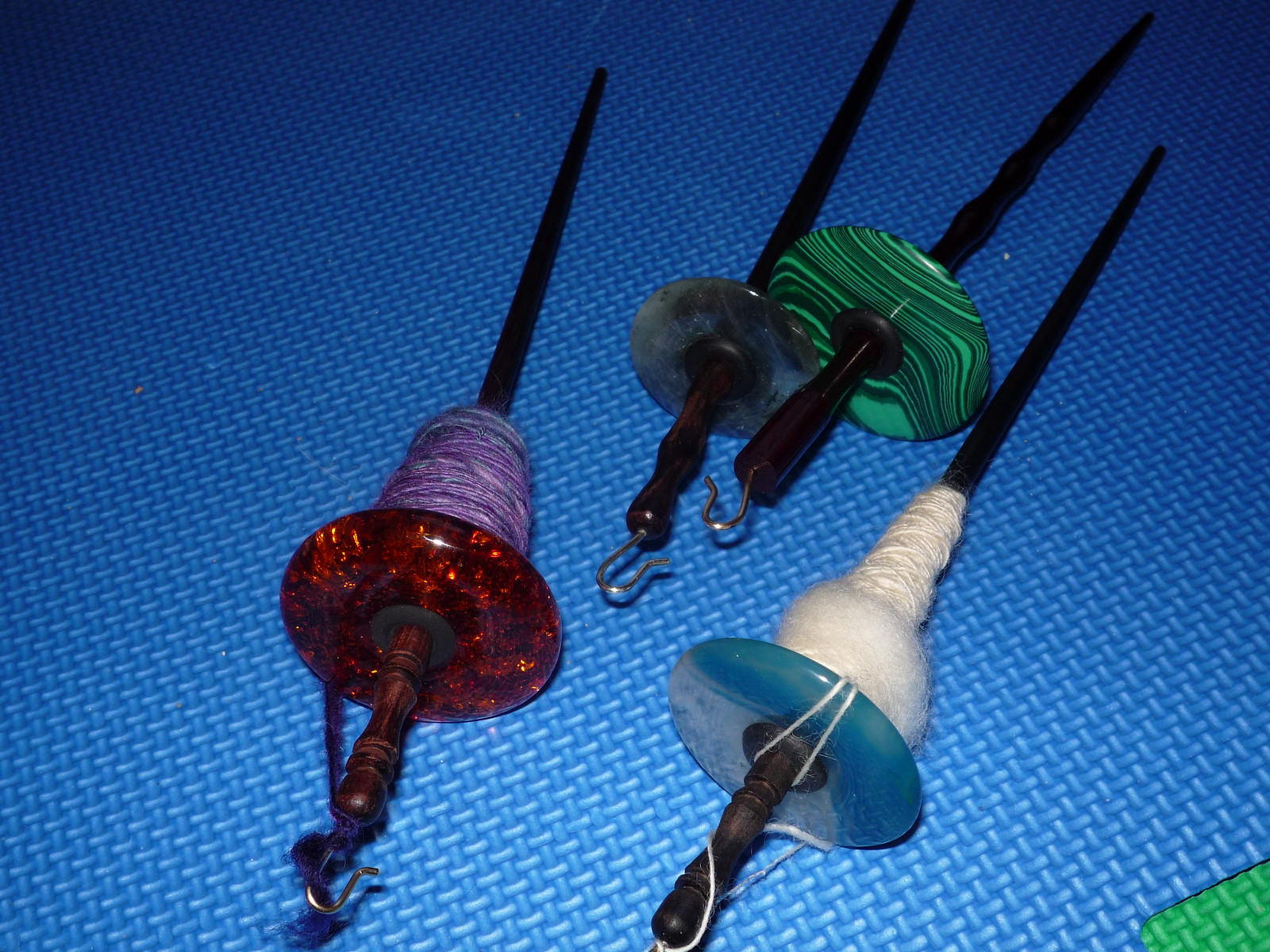This detailed image depicts four intricately ornate spindles, tools used for spinning, weaving, and winding threads. These spindles are positioned on a brightly lit blue and white textured foam mat, reminiscent of the interlocking mats often found in nursery schools. The mat appears to be made of colorful foam squares connected like jigsaw puzzle pieces, with a green section visible in one corner. Each spindle features a lathe-turned design with a disc-like platform or saucer, complete with a metal hook on the rounded end and a tapering point at the opposite end. The spindles vary in color and material, showcasing a range of beautiful hues and patterns: a deep metallic semi-transparent red that resembles lava, a green with marbling black swirls likely of malachite, an aqua seafoam blue akin to dyed quartz, and a clear bluish white one reminiscent of agate. Two of the spindles are wrapped with thread—one with purple and another with white—while the remaining two are bare. These spindles, possibly made from different stones like amber and malachite, are not only functional for textile work but are also highly decorative, making them captivating to look at.